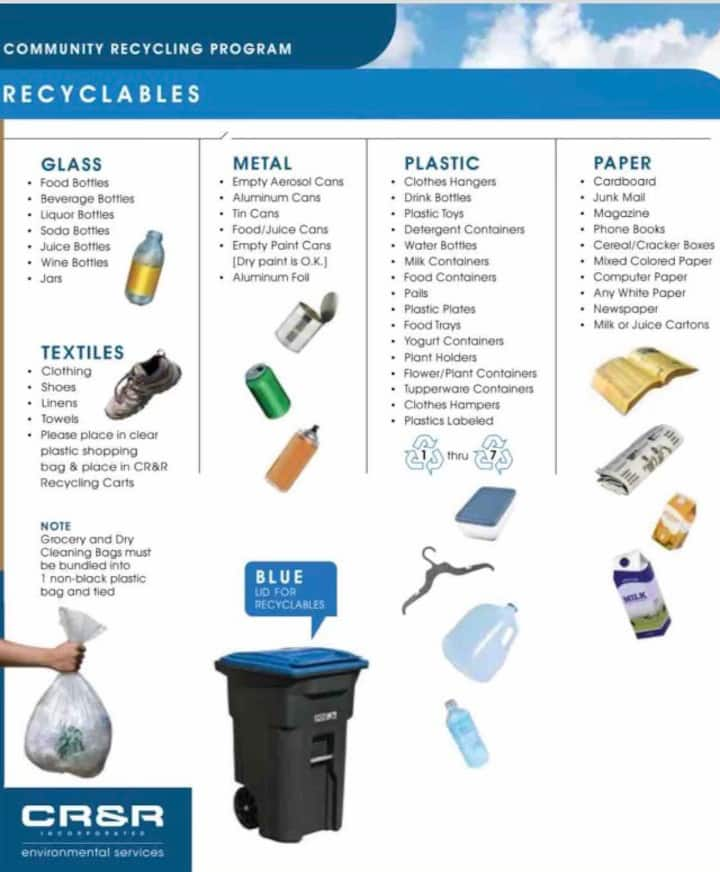This detailed infographic explains the Community Recycling Program, emphasizing recyclables. At the top, against a blue sky with clouds, a blue bar reads "Community Recycling Program" in white text, and a lighter blue bar below it states "Recyclables". The infographic is divided into four columns on a white background, each starting with a category name in blue: Glass, Textiles, Metal, Plastic, and Paper. Each category lists specific items that can be recycled, highlighted with bullet points. Under Glass, examples include food bottles, beverage bottles, and jars. The Textiles column lists clothing, shoes, and linens. Metal includes items like cans, while Plastic covers drink bottles, food trays, and yogurt containers. The Paper column mentions cardboard, junk mail, and magazines. The infographic also features images of these recyclables, such as a book, newspaper, milk carton, and more. At the bottom left, there is a CR&R logo, a black trash can with a blue lid, symbolizing recycling, alongside a trash bag and a Caucasian hand.